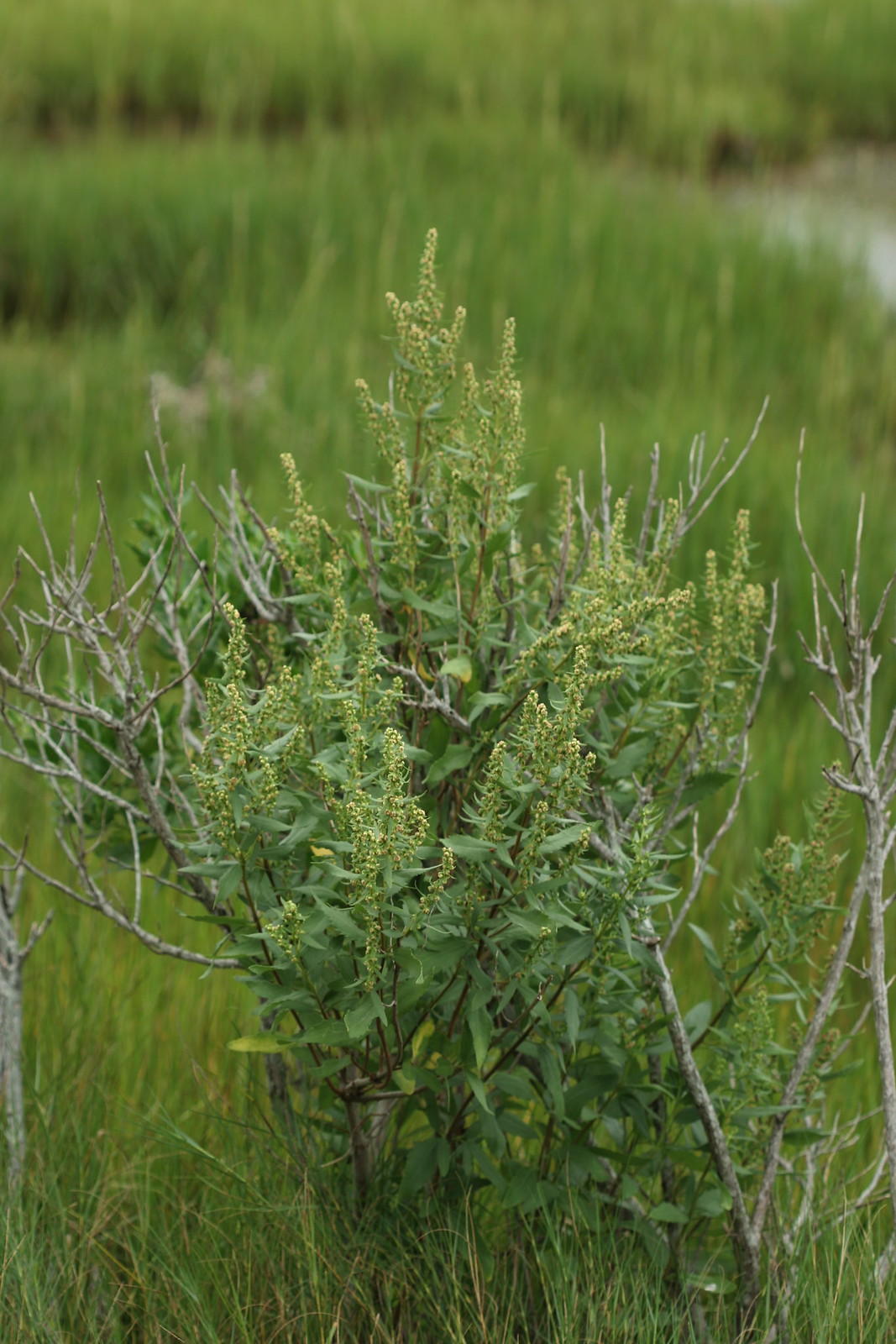This image features a large, weed-like plant in a grassy outdoor setting. The plant stands out with its long, green leaves resembling those of a mint plant. Toward the top, the plant has a light yellow flower that resembles wheat rather than a typical flower. Surrounding this focal plant is a stretch of normal green grass interspersed with a few twigs. In the background, similar grassy plants protrude from the ground, and there appears to be a small stream running through the scene, adding to the natural ambiance.